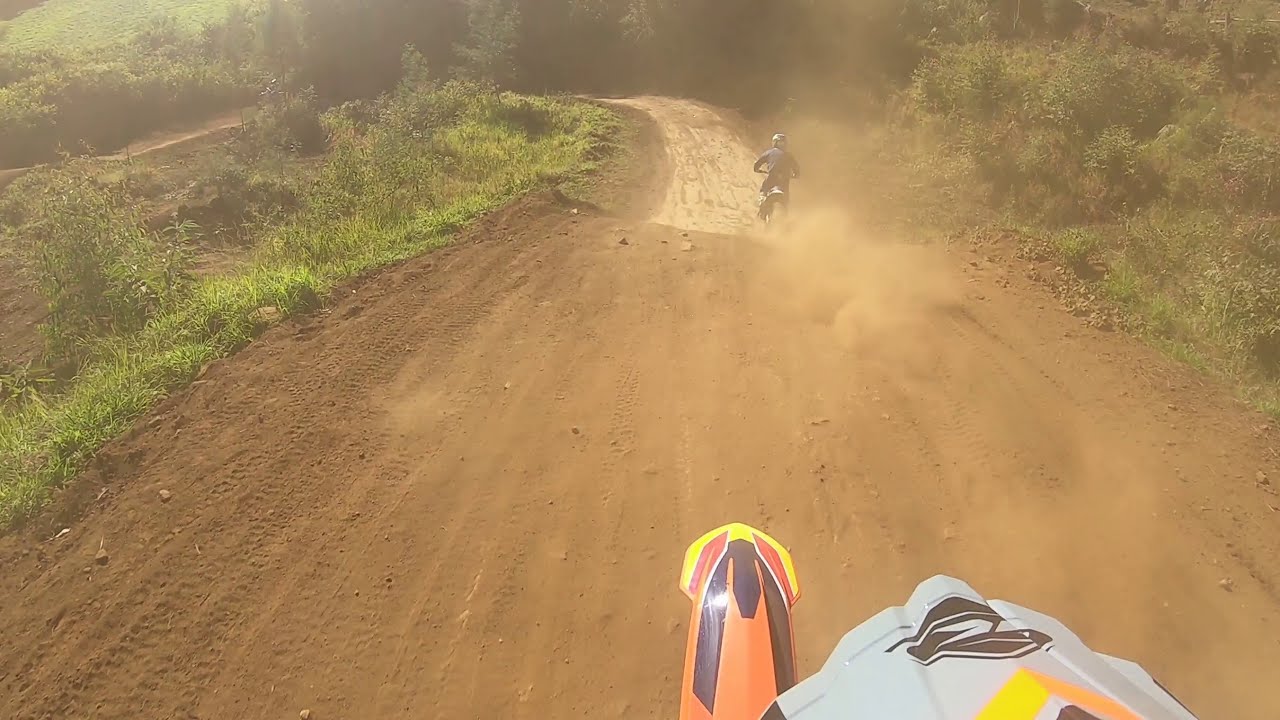In this image, we observe an outdoor scene set in the middle of the day on a wide dirt trail that runs vertically from the bottom center towards the top center. This dirt road, surrounded by a mix of green grass, bushes, and trees, serves as the setting for off-road motorcycling. On the trail, there are two motorcycles: one prominently in the foreground and another in the distance, both kicking up dust as they ride. The rider closest to the camera appears to be wearing a helmet possibly equipped with a mounted camera, as part of the motorcycle's front wheel guard is visible. The color palette includes earthy browns and tans of the dirt, the vibrant greens of the vegetation, and hints of orange, black, yellow, red, and gray from the motorbikes and surrounding features. There is no text present anywhere in the image.